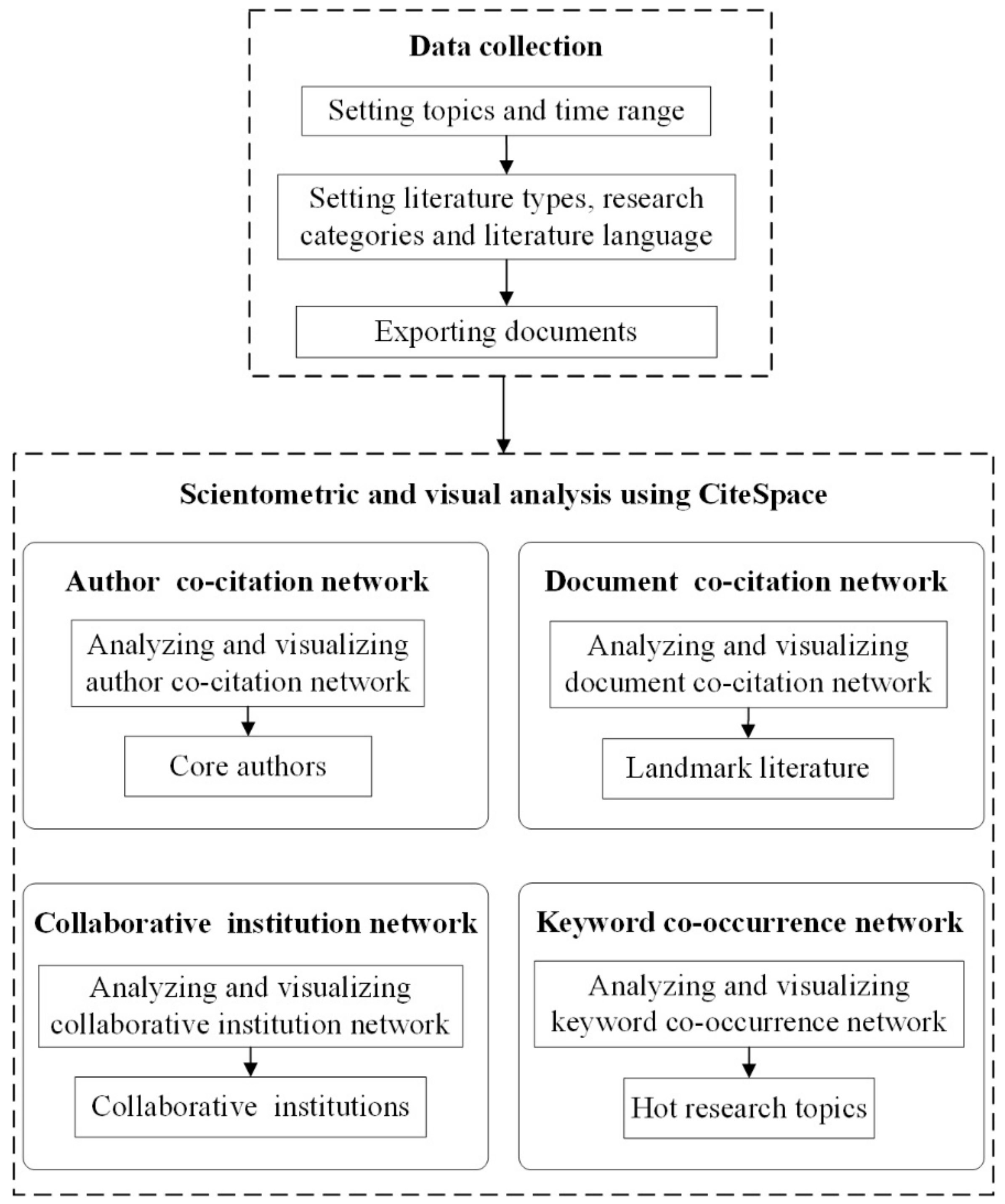Detailed and Structured Caption for Image:

The image depicts a procedural diagram framed by a dotted rectangular border. At the top, in bold Times New Roman font, the title "Data Collection" is prominently displayed. Below it, the diagram proceeds with multiple steps, starting with "Setting Topics and Time Range," followed by "Setting Literature Types, Research Categories, and Literature Language," and continues with "Exporting Documents."

Beneath this section, the diagram is divided into various analytical processes labeled as "Scientometric and Visual Analysis using CiteSpace." Subsections include:
1. "Author Co-Citation Network: Analyzing and Visualizing Author Co-Citation Network Core Authors."
2. "Collaborative Institution Network: Analyzing and Visualizing Collaborative Institution Network and Collaborative Institutions."
3. "Document Co-Citation Network: Analyzing and Visualizing Document Co-Citation Network Landmark Literature."
4. "Keyword Co-Occurrence Network: Analyzing and Visualizing Keyword Co-Occurrence Network."

Each subsection outlines specific areas of focus and methodologies for analyzing different dimensions of research data within the structured phases of data collection and analysis.